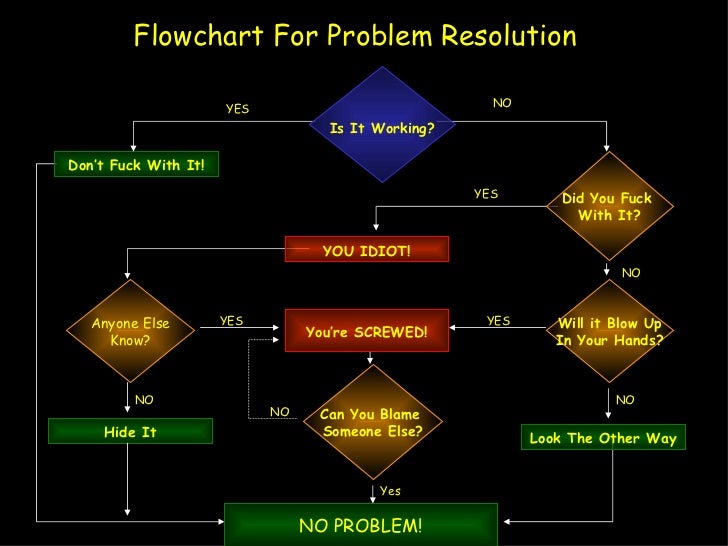### Flowchart for Problem Resolution

This humorous and profane flowchart, titled "Flowchart for Problem Resolution," is set against a dark or black background, with vibrant colored elements and text. At the very top is a blue diamond-shaped decision box labeled "Is it working?" If the answer is "Yes," an arrow leads to a green box with the blunt instruction "Don't fuck with it," which then guides you to the final resolution, highlighted in the bottom center: a green box labeled "No problem!"

If the answer to "Is it working?" is "No," the flowchart directs you to another decision box: "Did you fuck with it?" This box is light orange with yellow text. A "Yes" response from here leads to a red box stating "You idiot!" which then branches left to another decision diamond asking, "Anyone else know?" If "No," you are advised to "Hide it," leading back down to "No problem!" If "Yes," it goes to another red box saying "You're screwed," and then asks "Can you blame someone else?" If "No," it circles back to "You're screwed," creating a closed loop indicating inevitable failure.

On the "No" path from "Did you fuck with it?" the flowchart asks, "Will it blow up in your hands?" A "Yes" directs you immediately to "You're screwed," while a "No" leads to a green box advising you to "Look the other way," eventually resolving at "No problem!"

The overall design features diamonds and rectangles in blue, green, orange, and red, with arrows connecting each step in varied directions, emphasizing the comedic and chaotic nature of the chart.